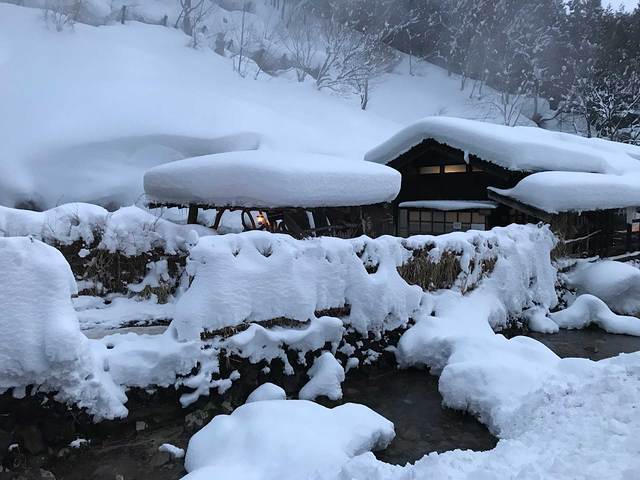In the photograph, taken at dusk, a large cabin sits on a snowy hill, enveloped in what seems to be a deep winter scene. The cabin, positioned to the right but central in focus, is blanketed with about one to two feet of snow on its roof and the canopy of a porch that extends out front. Next to the cabin, a carport or pavilion, heavily burdened with around three to four feet of snow, appears precarious. In the foreground, a snow-covered fence is nearly obscured under the weight of the recent snowfall. Beyond this, a frozen creek, its shallow waters mingled with snow and ice, stretches through the scene. The entire area suggests it is extremely cold, possibly near zero degrees Fahrenheit, with the surrounding hedges frozen over and seemingly lifeless. Despite the harsh conditions outside, the cabin emits a warm glow from its horizontal windows near the top, indicating the presence of electricity and a cozy refuge within. A small lantern is also lit under the snow-covered gazebo, further emphasizing that the inhabitants are nestled inside, secure from the freezing elements.